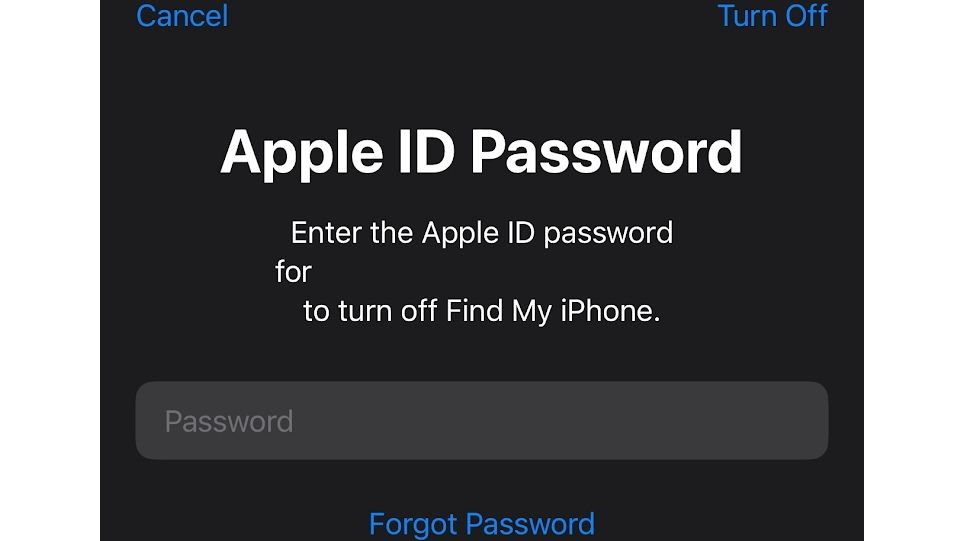The image displays a user interface for entering an Apple ID password to disable the "Find My iPhone" feature. The background is primarily black.

- In the top left corner, there’s a blue text saying "Cancel."
- In the top right corner, there’s a blue text saying "Turn Off".

Centered below these options, in bold white text, is the phrase “Apple ID Password”. Directly underneath, in slightly smaller and less bold white text, is the instruction to "Enter the Apple ID password for to turn off Find My iPhone."

Below this instruction, there is a gray rectangle with rounded corners, containing the text "Password" in a lighter shade of gray.

At the bottom of the interface, there’s a blue text saying "Forgot password."

The high contrast between the boldness and colors of the text elements emphasizes the primary action of entering the password and the secondary options available.